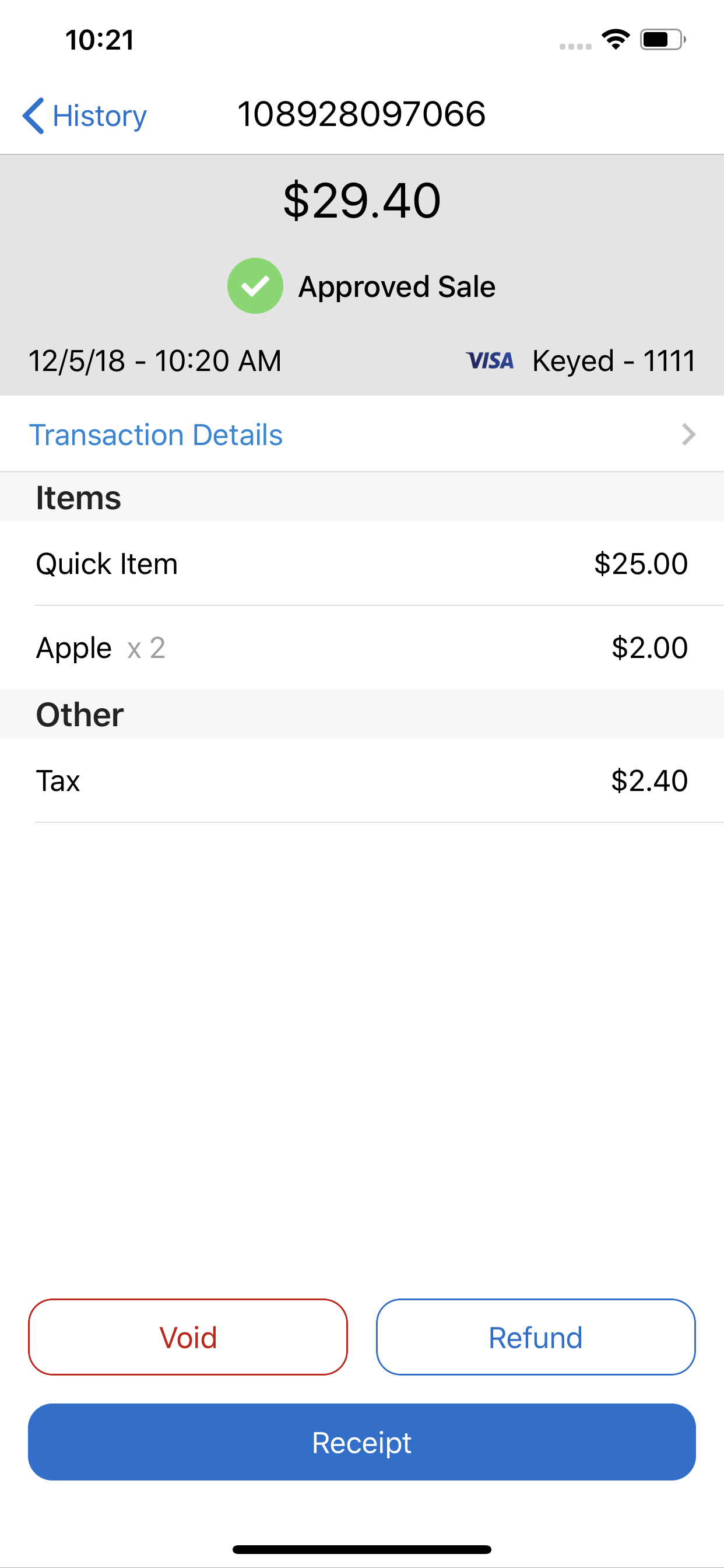This mobile screenshot captures a merchant payment app screen detailing a recent transaction. At the top left corner, the word "History" is displayed in blue font, accompanied by a leftward arrow for navigation. Centrally positioned at the top, we see the transaction's sale number in black font. 

Directly below the sale number, a large gray box prominently displays the total amount of "$29.40" in big black numbers. Beneath this amount, the text "Approved Sale" appears centered, with a green circle and white check mark icon to the left, indicating the transaction's approval status. At the lower left corner of this box, the date and time "12/5/18 10:20 a.m." are noted. On the right side, the Visa logo appears, marked as "keyed" with the number sequence "1111."

The background following this section is white, featuring "Transaction Details" in blue font at the top left, with a rightward arrow on the far right for expanding more details. Below is a gray bar labeled "Items" in bold black letters. The itemized list includes:
- "Quick Item: $25
- "Apple (x2): $2
- "Other: --"
followed by "Tax: $2.40."

At the bottom of the screenshot, there are three buttons: a red "Void" button on the left, a blue "Refund" button in the center, and a large blue "Receipt" button spanning from left to right at the bottom.